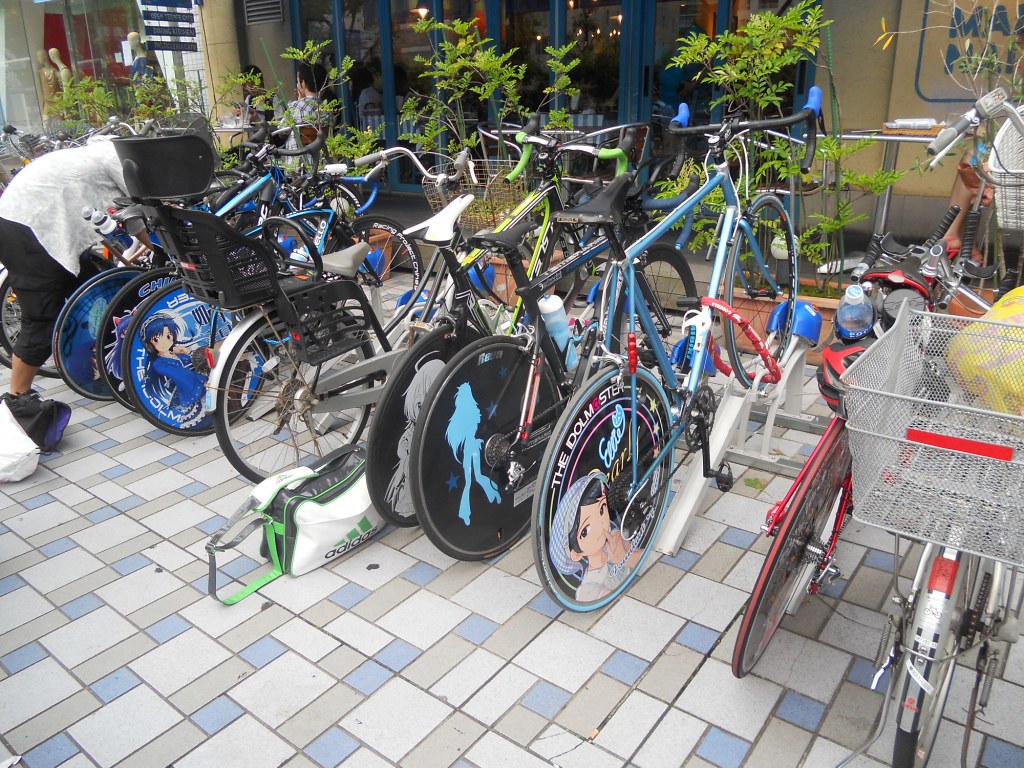The photograph depicts an outdoor scene seemingly set in a shopping area or outdoor mall, during daytime hours. The ground in the image is covered with tiles arranged in squares and rectangles, featuring off-white, gray, and sky blue colors. This tiled mosaic floor serves as the base for a clutter of bicycles, roughly about ten in total, parked within a bike rack. The bikes are varied in size, style, and color, many showcasing thin tires and anime character designs, predominantly of female characters, on their rear wheels. Among the assortment, there is a bike with a basket located at the bottom right and another with a seat for an extra passenger. Alongside the bicycles, there is a white-and-green traveling bag near one of them, and a person dressed in a white shirt and black pants is visible in the top left corner, possibly interacting with their bike. The scene is set against a backdrop of a blue-colored shop with windows, and there is a thin line of mid-sized, feathery green plants acting as a barrier between the tiled bike area and the shopfront.